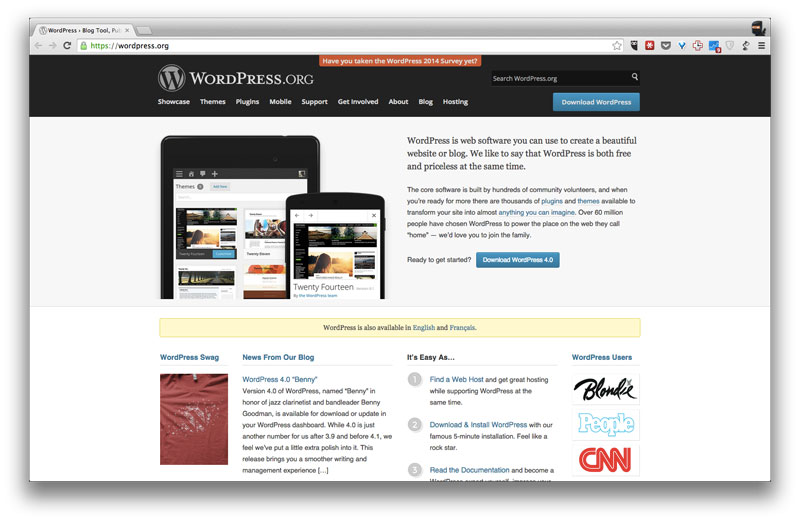This screenshot depicts the WordPress.org homepage, highlighting their 2014 survey with a prompt, "Have you taken the WordPress 2014 survey yet?" prominently displayed. The site’s header features the WordPress logo, a stylized "W" in a gray circle on a black background, with navigation options for Showcase, Themes, Plugins, Mobile Support, Get Involved, and more, aligned horizontally.

Central to the screenshot is a blue (almost teal) button labeled "Download WordPress," accompanied by the text: "WordPress is web software you can use to create a beautiful website or blog. We like to say that WordPress is both free and priceless at the same time." This description underscores the platform's value and accessibility, further emphasized by visual representations of WordPress on both a tablet and a smartphone, with a call-to-action text, "Ready to get started?"

Below, a yellow notification box indicates that WordPress is available in English and French, with the word "Français" accentuated for clarity. 

A featured image later on the page shows a swatch of material embedded with glass-like items, promoting "WordPress swag." This section introduces WordPress 4.0, whimsically named "Benny" after jazz legend Benny Goodman. It assures users of added polish in version 4.0 while maintaining its numerical sequence between 3.9 and 4.1.

To the right, step-by-step instructions, titled "As easy as 1, 2, 3," guide users through finding a web host, conducting WordPress’s famous five-minute installation, and reading the documentation, with a tongue-in-cheek reference to "Blondie" at step one.

Overall, this screenshot offers a detailed overview of the WordPress.org homepage, emphasizing its accessibility, multistep simplicity, and the new features in the 4.0 update.